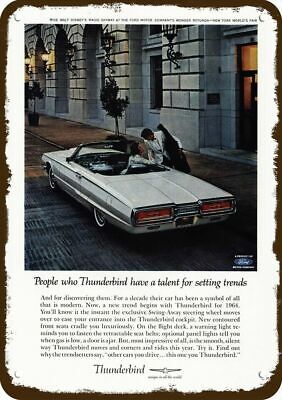The image depicts a vintage advertisement styled like a collectible trading card for a classic Thunderbird convertible. The ad features a tiny, color photograph framed by a jagged dark border, showing a sleek, white Thunderbird car with its top down, parked in front of a large, gray stone building, possibly indicating an upscale street setting in the evening. The focus of the picture is on a man in a white tuxedo jacket and black tie, who appears to be a parking attendant, leaning over to talk to a woman seated in the passenger seat. The woman, dressed in a white, long-sleeved top, and the man’s actions suggest he is either helping her out of the car or preparing to park it. The headline at the top of the ad reads, "People Who Thunderbird Have a Talent for Setting Trends," echoing a stylish and trendsetting theme. Below the image, there’s a block of text in small font, and at the bottom, the brand name "Thunderbird" along with its logo is prominently displayed. The card itself has a distressed light brown border, enhancing its vintage appeal.